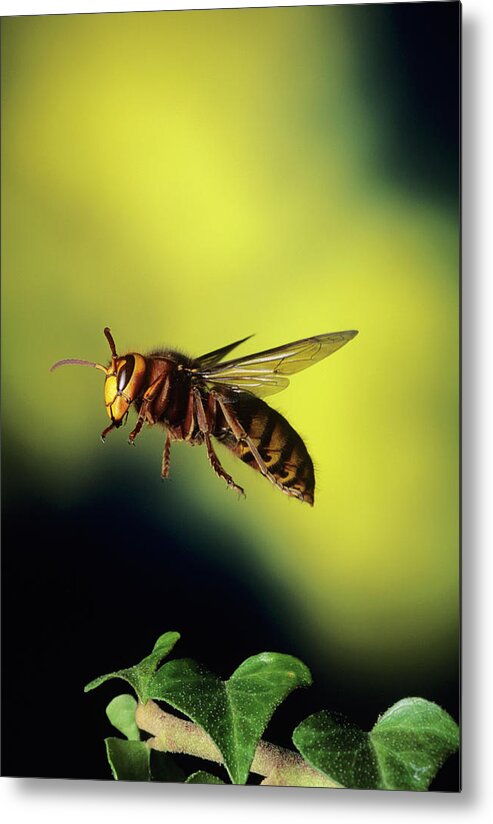This striking photograph captures a Hornet in mid-flight, prominently displayed against a vibrant and slightly blurry green background. The Hornet, with its yellow head and black eyes and antennae, exhibits a distinctive pattern of yellow and black stripes on its abdomen. The wings are outstretched, showcasing their transparent nature. Notably, the photograph reveals intricate details such as the tiny bristles on its feet and legs, as well as the fuzz on its thorax. Below the Hornet, delicate, heart-shaped green leaves add a touch of natural beauty to the composition. The overall effect is a vivid, eye-catching image that emphasizes the Hornet's vibrant colors and detailed anatomy.